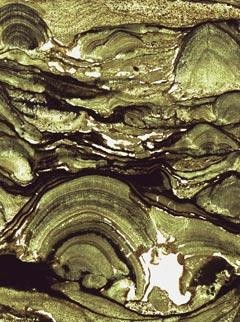The image showcases a close-up view of a complex and layered rock formation with a greenish cast interspersed with blacks, yellows, and browns. This rock, which has a glossy appearance that could be attributed to the lighting or the reflective nature of the surface, displays multiple layers and compressed arcs suggesting geological formation over centuries. The texture appears uneven, with rough layers that evoke the shape of fossilized or polished oyster shells, adding to the enigma of its origin. In the bottom part of the image, a striking white spot stands out, giving off a glow that might be light reflection or a mineral inclusion. This area also features chips and irregularities, as if the rock has been fractured, exposing its intricate internal structure.